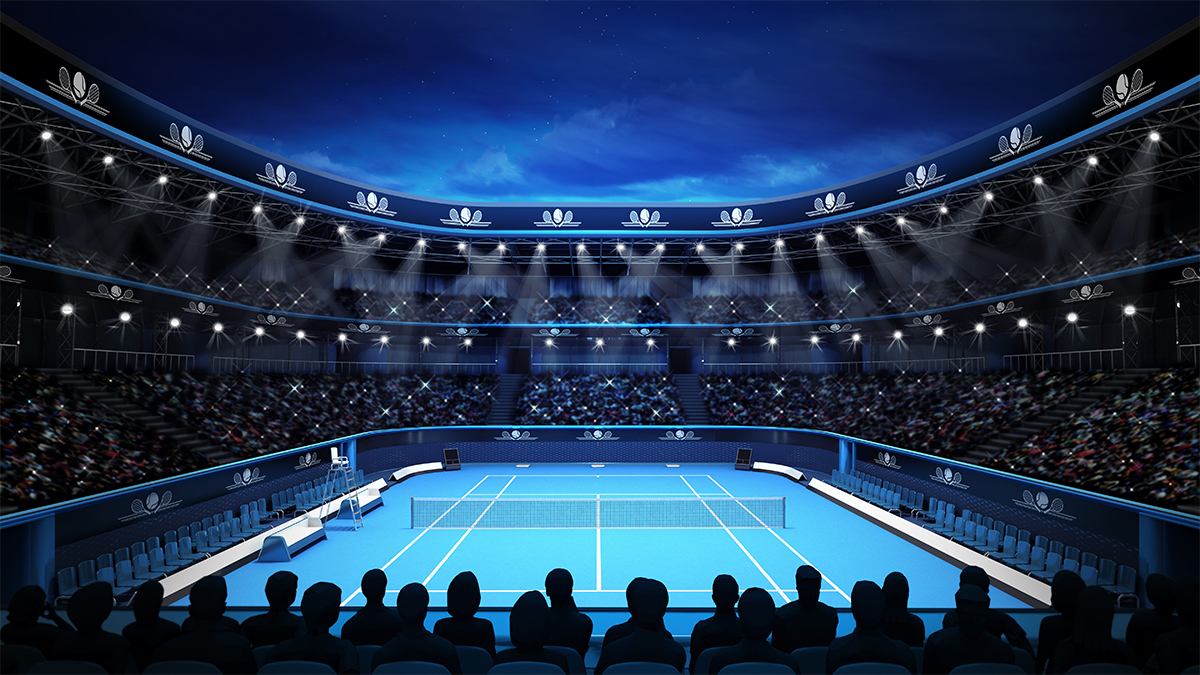This detailed image captures a 3D-rendered, semi-realistic tennis stadium with a somewhat futuristic design. The stadium is an open, two-tiered oval structure bustling with spectators whose individual features are not discernible. The tennis court at the center is light blue, transitioning to darker blue towards the edges, and marked with white lines. On either side of the court, there are designated seating areas for players fitted with blue chairs, with decorative white borders surrounding these areas. An elevated seat for the referee is noticeable on the left side, while overhead, lights encircle the top level, illuminating the court below. The open roof reveals a dark blue, cloudy night sky, adding to the overall clean and animated feel of the scene. Additionally, a logo featuring two tennis rackets and a tennis ball decorates the stadium, emphasizing its animated and video game-like appearance.